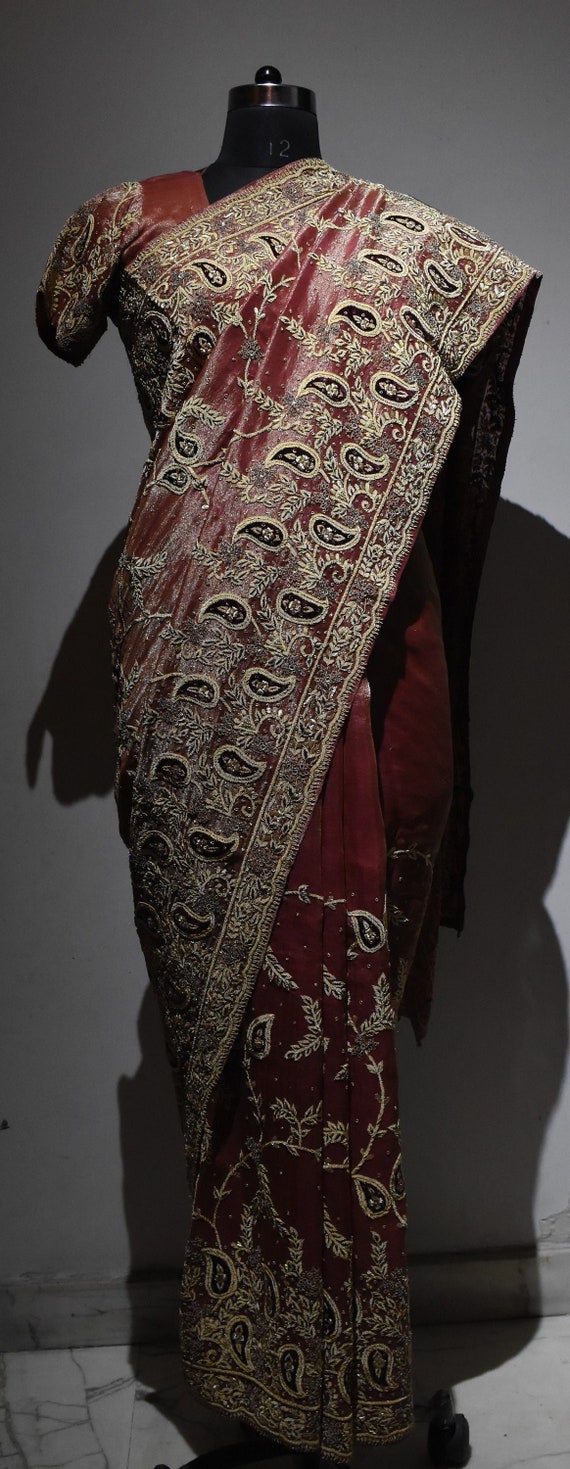This photograph captures a traditional Indian outfit displayed on a headless black mannequin, set against a dark, gray background with a marble floor. The attire appears to be a sari, featuring a short-sleeved blouse and a long, elegant fabric wrap. The ensemble is predominantly a deep wine or burgundy color, lavishly adorned with intricate gold paisley, leaf, and fern-like patterns. The sari is intricately draped over the right shoulder, while the short sleeve is visible on the left, with the flowing fabric nearly reaching the floor. The material has a high sheen, adding a lustrous quality to the entire outfit. Notably, the number "12" is placed on the mannequin, possibly indicating a size or exhibit number. The overall setting suggests a museum display, underscored by the ambient lighting and dark shadows that enhance the visual impact of the traditional costume.